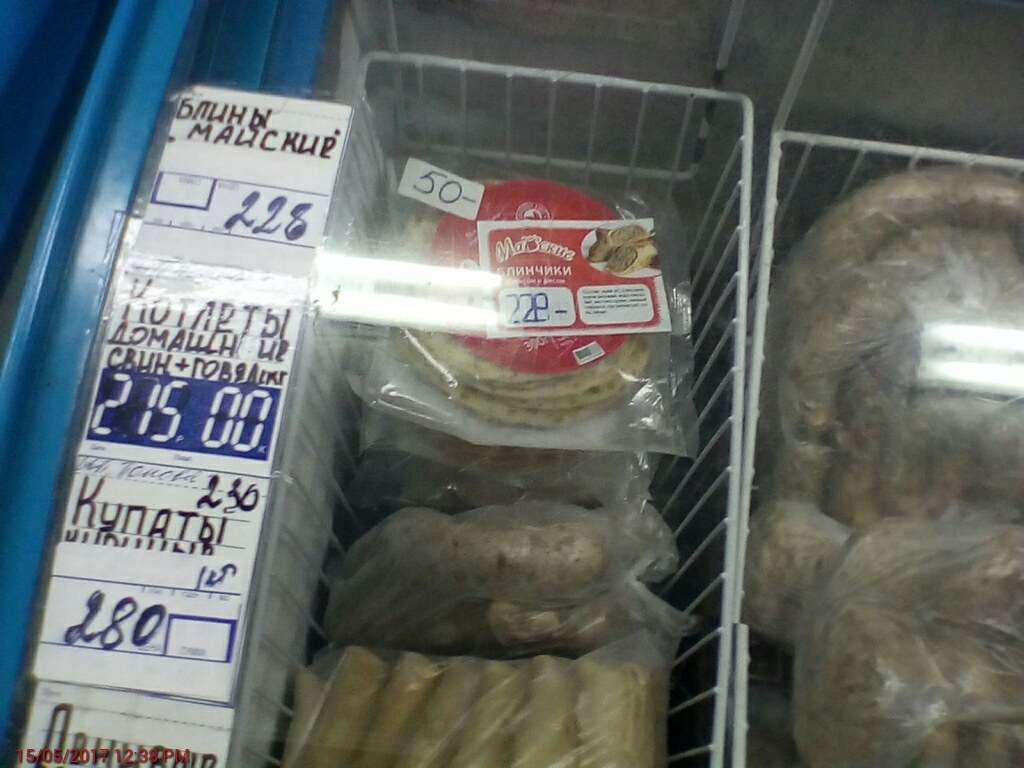This photograph appears to capture a section of a market or store, featuring a couple of metal racks or baskets within what seems to be a freezer or cooler. On the left side of the image, a distinct blue metal border runs diagonally from the bottom left corner towards the upper right, exiting the frame at the top. Affixed to this border is a white sticker with some unintelligible text and a series of numbers: 50, 228, 230-280, possibly indicating prices or other information. 

Alongside the blue border, towards the right, there are two metal racks. The first rack is partially visible and holds various food items, which appear to be frozen and wrapped in plastic. The top shelf contains what might be frozen pancakes, followed by shelves with sausages and perhaps burritos. The adjacent metal rack, about 80% visible and extending off the right edge of the image, also contains food items, mainly large plastic bags filled with sausages. 

Additionally, the photograph captures a date and time stamp in red at the bottom, stating: "May 15, 2017, 12:38 PM." The overall setup suggests a refrigerated display area within a market, organized with assorted packaged foods such as tortillas, meat, tacos, beans, and potatoes.